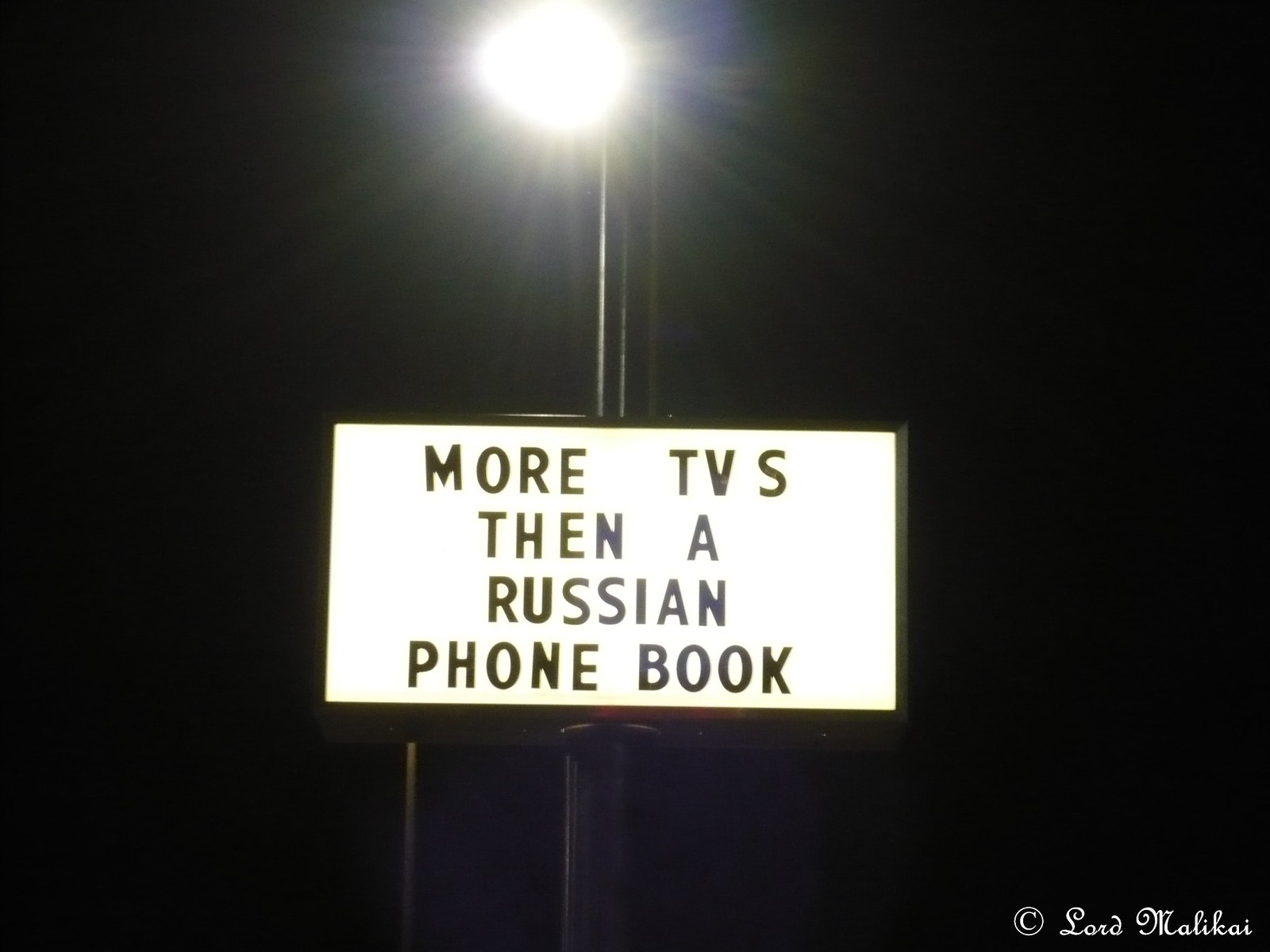In this nighttime photograph, the scene is set against a backdrop of a pitch-black sky. The focus is on a tall metal pole that supports both a lit-up street light at its pinnacle and a white marquee beneath it. The street light glows brightly, casting a stark contrast against the dark surroundings. The marquee is prominently displayed, featuring bold black letters that spell out the message: "more TVs then a Russian phone book," with a noticeable typo, as "then" should be "than". In the bottom right corner of the marquee, in elegant white cursive, is the signature "Lord Malachi," accompanied by a circled "C" indicating copyright. The overall illumination highlights the marquee’s details while leaving the surrounding environment shrouded in darkness.